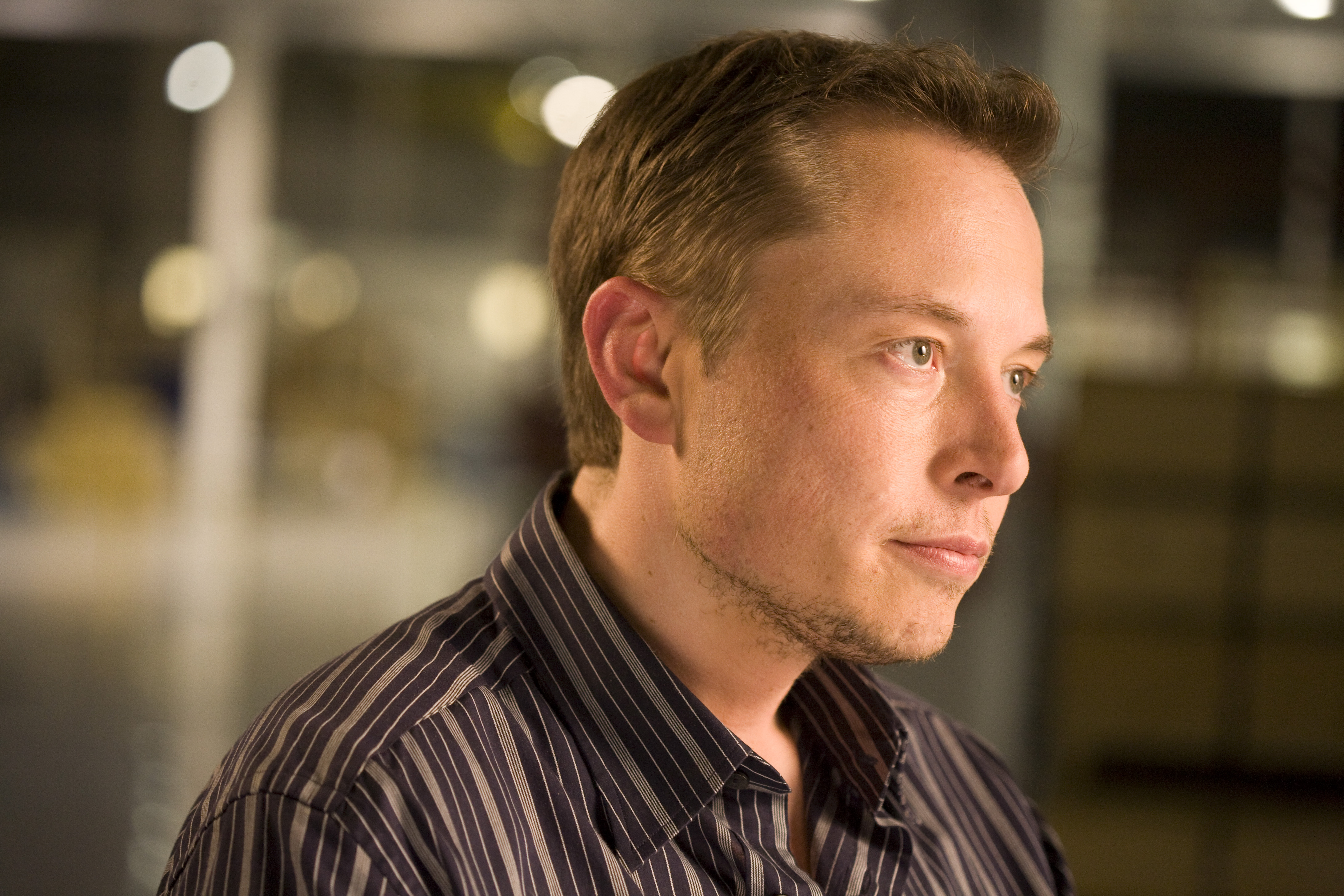In this photograph, a younger Elon Musk is captured with light brown hair and matching light brown eyes. His hair is relatively short, though a bit scruffy under his chin, accompanied by a slight beard and mustache. Musk is gazing intently but politely to the right, likely at an interviewer. He wears a taupe and dark grey striped button-up collared shirt. The image, wider than it is tall, only shows him from the top of his chest and shoulders upward. The background is blurred with fuzzy lights, revealing some colors such as yellow, blue, brown, black, and beige, indicating he is indoors. There's a light shining on his head, and he holds a virtually expressionless demeanor, different from the more familiar Elon Musk of today.